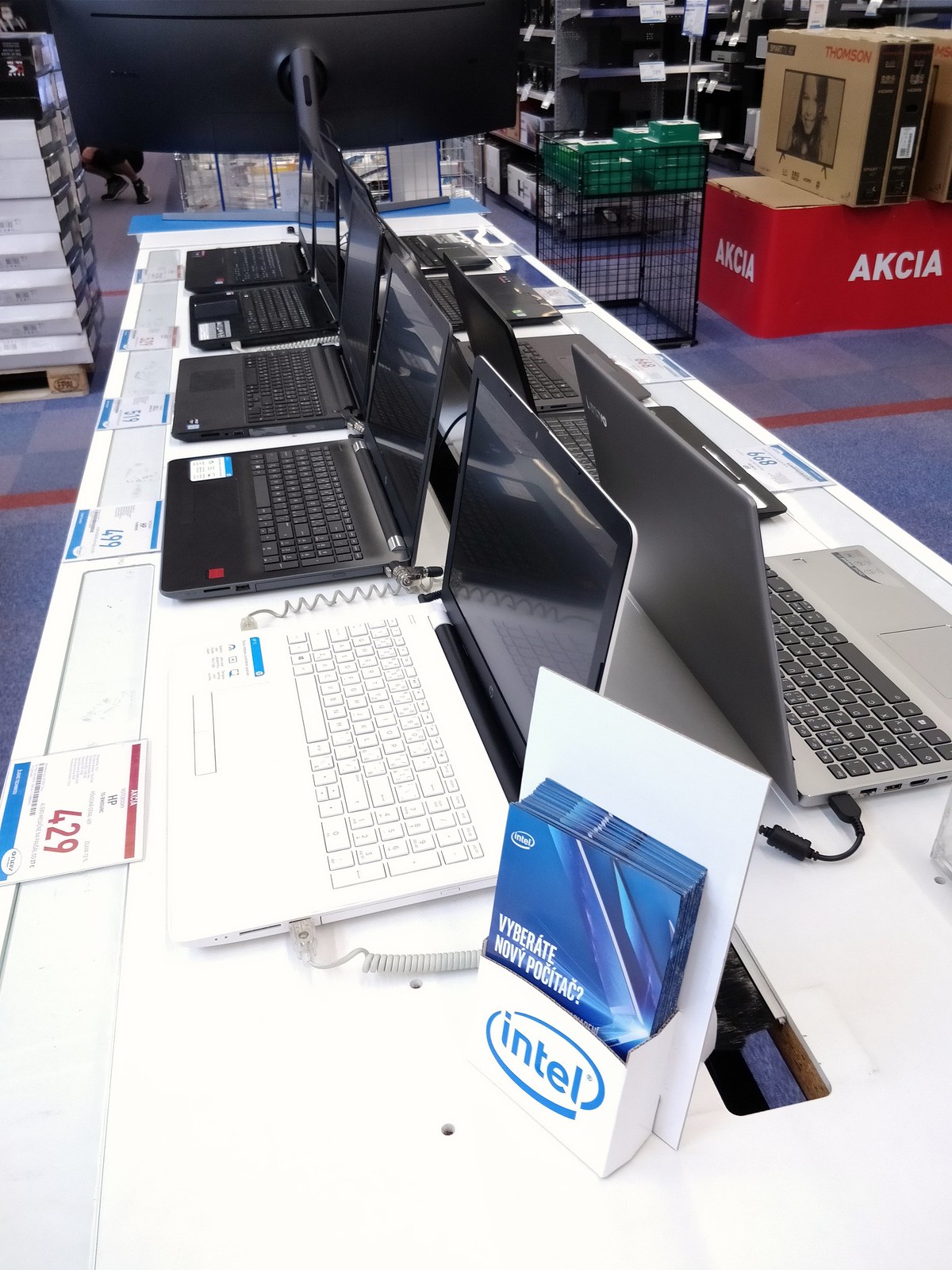The color photo showcases the bustling atmosphere of an electronics store, possibly a Best Buy or Staples. Dominating the foreground is a large table adorned with ten open laptops arranged in two back-to-back rows. Most laptops are sleek black or dark gray, except for one standout white model positioned at the bottom left, priced at $429. The setup includes a prominent black monitor at the top and a display stand featuring blue Intel brochures with white text. A vivid background filled with tools, stacks of materials, and built-up red displays adds to the store's busy ambiance, emphasizing the array of electronics on offer.